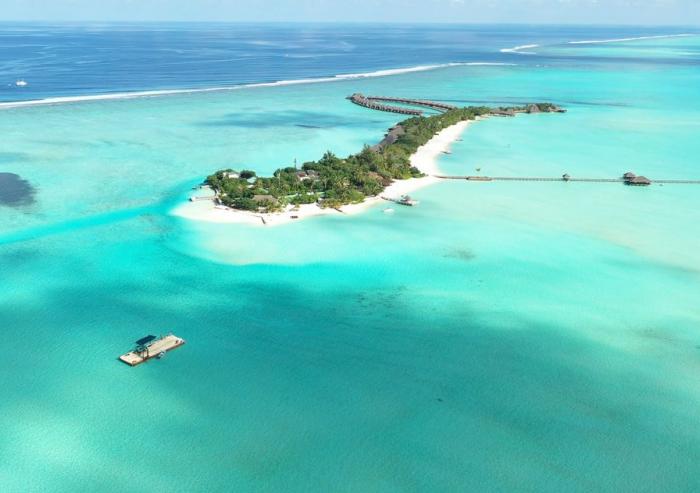In this aerial landscape photograph, a picturesque tropical island is depicted, surrounded by serene, multi-hued waters that range from deep blue to seafoam green. The central focus of the image is a small, lush atoll with a distinct, white sandy beach that creates an S or J-shaped contour around the greenery. Tall trees and scattered houses are seen dotting the island, which is further enhanced by numerous piers extending into the vibrant, clear blue-green ocean.

Starting from the island's center, a long pier stretches out towards the horizon, flanked by two structures: a smaller one midway and a larger one at the far right, notable for its visible roof. A unique, circular pier with numerous connecting paths and several thatched huts suggests a luxurious resort destination. To the bottom left of the photograph, a flat-roofed boat with a person aboard can be seen, accompanied by two small rafts moored to a tiny floating pier.

The sky forms a crisp, bright blue backdrop that seamlessly merges with the captivating hues of the ocean. The scenic beauty and intricate layout imply a tranquil vacation spot rich in natural charm and recreational opportunities, framed by the open expanse of sky and sea.